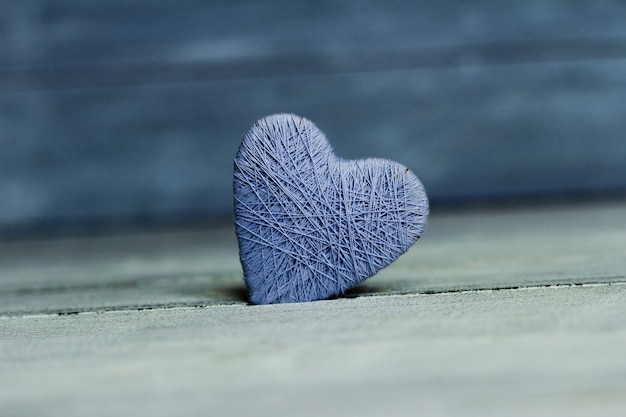The image is a detailed, color photograph featuring a heart-shaped form wrapped in an intricate network of dark gray, blue, and lavender strings. The heart appears to be crafted meticulously, with hundreds of meters of string crisscrossing and binding it. It is tilted to the right and wedged into a crack within a rough, dry, grayish wooden floorboard. The heart casts a shadow on the floor, adding depth to the scene. The background is blurry, featuring a dark bluish, slate-gray color, possibly wooden paneling, creating a bokeh effect that keeps the heart in sharp focus while everything else appears hazy. The overall color palette of the photograph includes shades of gray, blue, and lavender, enhancing the surreal, almost computer-generated aesthetic of the image.